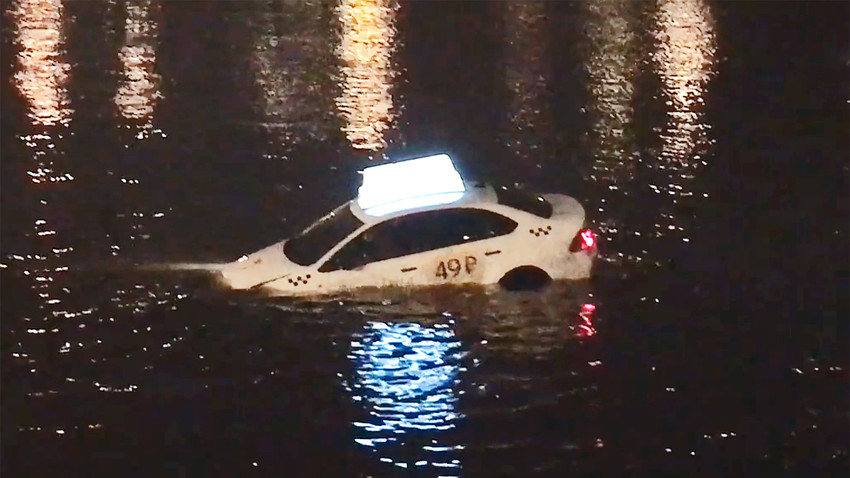The image depicts a white car, likely a taxi or delivery vehicle, sinking in a large body of water at night. The scene suggests an urban setting, inferred from the reflections of city lights on the water’s surface. The car has a lighted sign atop it, though the specific text is not readable. It displays a number "49P" on the rear passenger door, along with black and white checkered patterns near the front and back. The car is at approximately a 30-degree angle, with the front deeply submerged and the rear starting to follow. The front tires are almost completely underwater, while the back tires are only partially submerged. The car's headlights and brake lights are on, creating a stark illumination in the dark water. Reflections from other city lights add more brightness to the scene, casting patterns on the water.